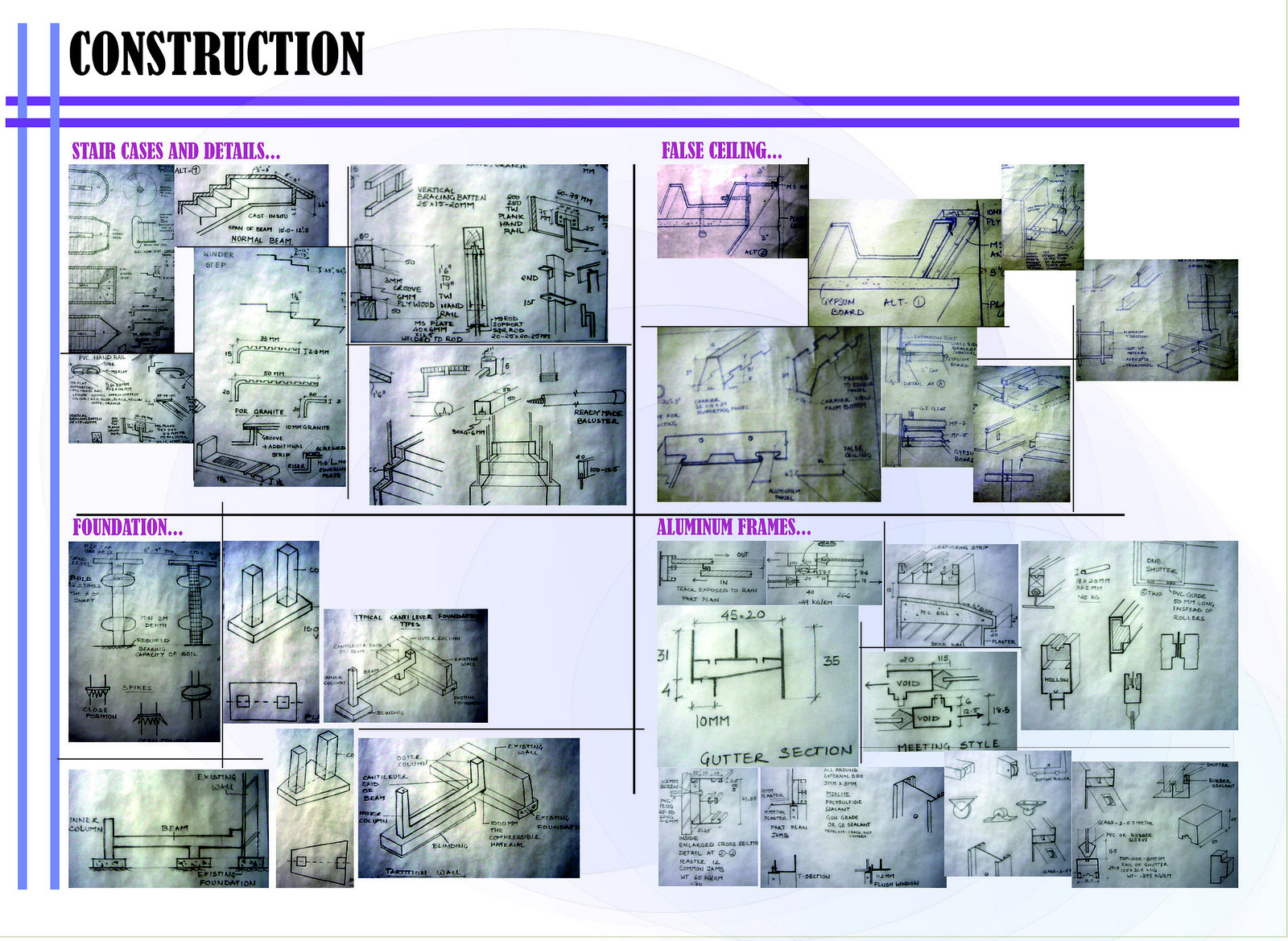The image appears to be a scanned construction schematic divided into four neatly organized sections, each featuring detailed plans related to various aspects of construction. The upper left corner has the word "CONSTRUCTION" prominently displayed in bold, black uppercase font. Surrounding this are intersecting purple lines that form a grid structure, creating a visually framed layout.

Each quadrant of the grid showcases specific construction elements:
- **Upper Left (Staircases and Details):** Contains six meticulously hand-drawn blueprints focusing on staircase designs and detailed measurements.
- **Upper Right (False Ceiling):** Features seven detailed schematics outlining the plans for installing false ceilings.
- **Lower Left (Foundation):** Displays six detailed, hand-drawn plans elaborating on the foundation construction process.
- **Lower Right (Aluminum Frames):** Includes ten drawings illustrating the construction and installation of aluminum frames.

Text labels for these sections are written in purple, providing clear and organized headings that differentiate between the various construction components. The overall image is a comprehensive, visually organized collection of construction plans, meticulously detailed to guide the construction process.